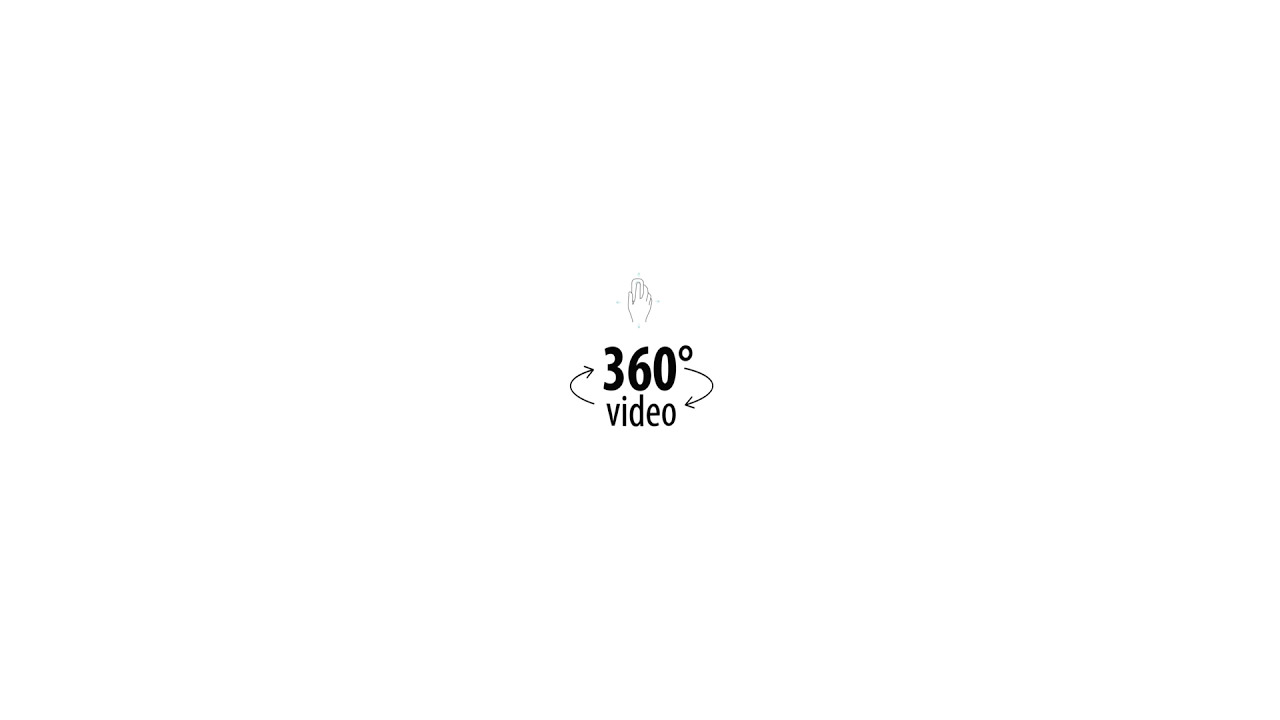In the image, there is a completely white background that blends seamlessly with the rest of the computer screen. Centrally positioned, there is a small icon roughly the size of a pencil eraser, depicting the outline of a right hand holding an oval-shaped object, likely a mouse. The thumb is on the left, the index finger is on top, and the remaining fingers are curled around the object, with the wrist area open. The hand is outlined in a light shade of black, providing subtle contrast against the white backdrop.

Below the hand, the text "360°" is boldly printed in black, and directly underneath that, the word "video" appears in a thinner, dark black font. Additionally, there are two arrows: one on the left side of the hand that loops from the word "video" to point towards "360," and another on the right side that extends from the degree symbol in "360°," curving downward to point back up towards "video." The minimal use of colors—primarily white, black, and a hint of gray—and the central placement of the icon and text suggest it might be a logo, potentially suited for a stock image website.